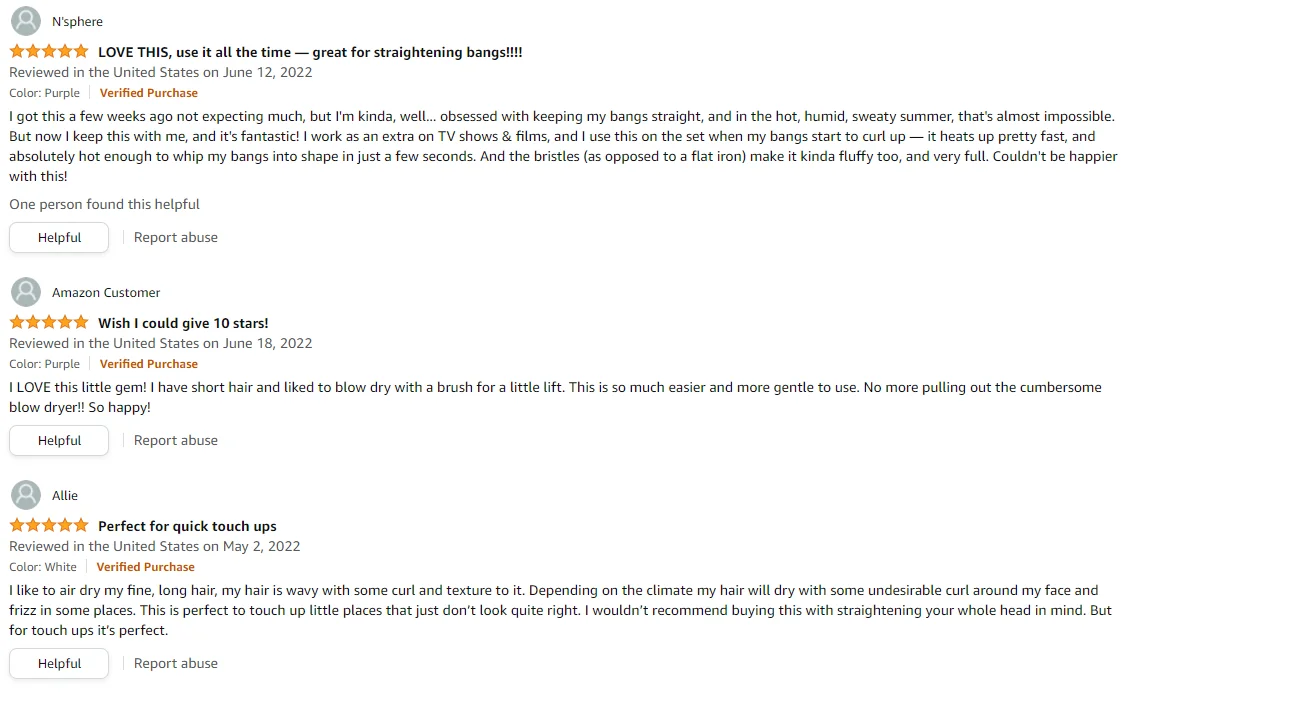The background of the image is white. It appears to be a screenshot taken from the review section of a product page on Amazon, with Vietnam in the product name. The image includes three detailed customer reviews:

1. **User: NSPIR (Rated 5 Stars)**
   - **Caption:** "Love this, use it all the time! Great for straightening bangs. I got this a few weeks ago without expecting much, but I've become obsessed with keeping my bangs straight, which is almost impossible in the hot, humid, sweaty summer. Now, I can carry this with me, and it's fantastic. I work as an extra on TV shows and films and use this on set when my bangs start to curl up. It heats up pretty fast and is hot enough to whip my bangs into shape in just a few seconds. Unlike a flat iron, the bristles make my bangs fluffy and full. Couldn't be happier!"

2. **User: Amazon Customer (Rated 10 Stars, metaphorically)**
   - **Caption:** "Wish I could give ten stars! I love this little gem. I have short hair and enjoy blow-drying it with a brush for a bit of lift. This tool is so much easier and gentler to use—no more dragging out the cumbersome blow dryer. I'm so happy with this purchase!"

3. **User: Allie (Rated 5 Stars)**
   - **Caption:** "Perfect for quick touch-ups. I like to air-dry my fine, long hair, which is wavy with some curl and texture. Depending on the climate, my hair sometimes dries with undesirable curls around my face and frizz in some spots. This tool is perfect for touching up those little areas that just don't look quite right."